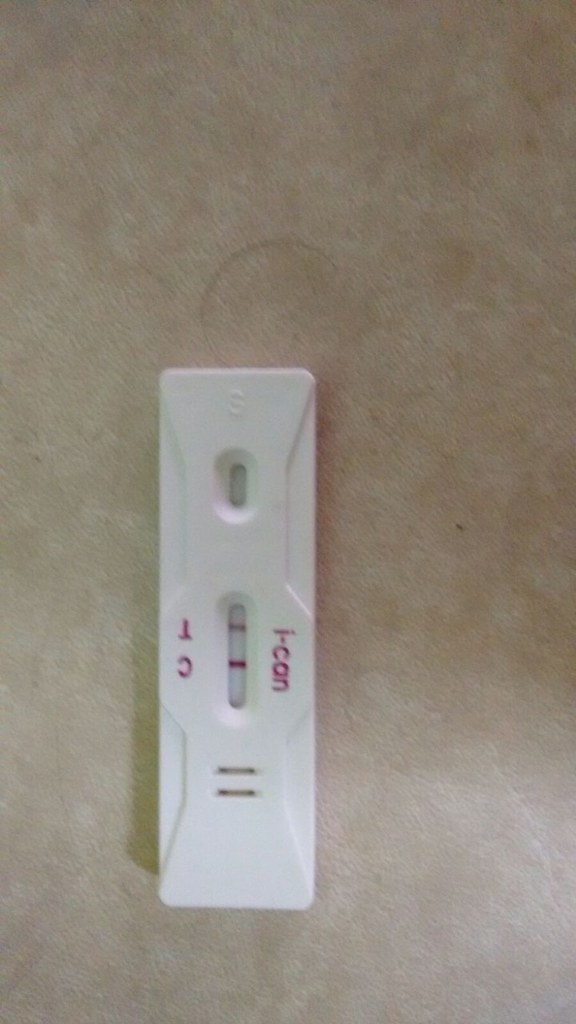This image is an aerial photograph of a small white rectangular device, likely a COVID-19 test kit. The test kit features a three-dimensional design with a noticeable oval-shaped groove at the top, intended for the application of testing drops. Below this groove is a longer, rounded rectangular section with two distinct pink lines—one slightly thinner than the other. To the left of these pink lines, there are markings that resemble an upside-down "T" next to a backwards "C." To the right, the text "I-can" is visible. Additionally, the center of the device features two small dashes positioned horizontally, resembling an equal sign. The test kit rests on a tan-colored surface, possibly a table or countertop, which serves as the background for the photograph.